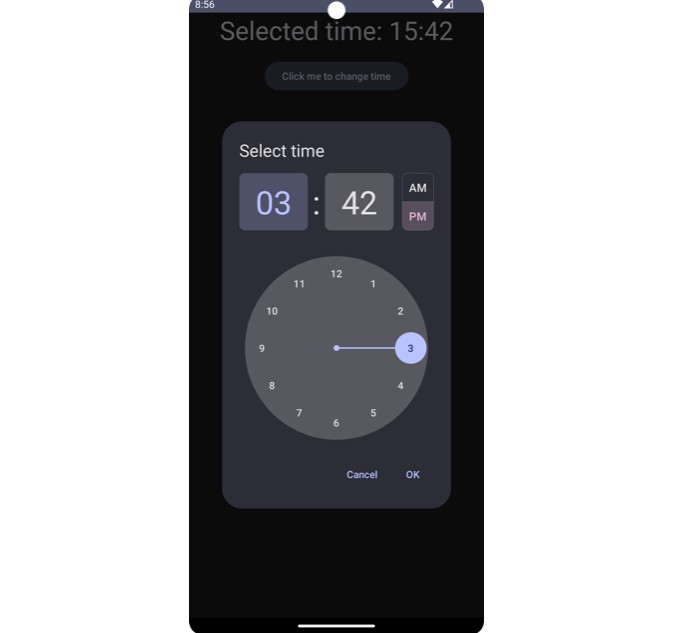The image is a screenshot of a cell phone screen displaying a user interface for setting the time. The background of the screen is solid black, which contrasts sharply with the interface elements. At the top, there is a small section with the text "Selected Time: 15:42." Directly beneath this text, there is a gray-colored button labeled "Click me to change time."

The central feature of the screen is a prominent, lighter gray box that occupies most of the middle area. In the upper left corner of this box, the text "Select Time" is displayed in white font, with a capitalized "S". Below this heading are two input fields: the first one is for selecting the hour, and the second one is for selecting the minutes. To the right of the minutes box, there is an additional selection box for choosing between "AM" and "PM."